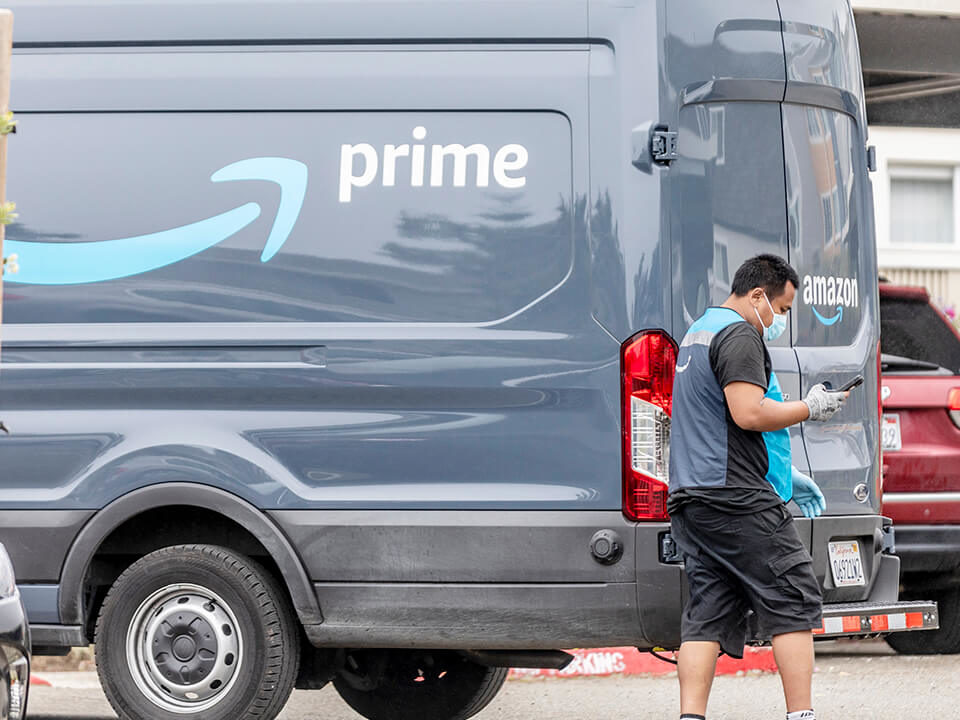A detailed image captures the rear half of an Amazon Prime delivery van, parked outdoors. The van is a dark blue color, prominently displaying the Prime logo in a striking teal blue and the brand name Amazon in bold white lettering. An Amazon Prime worker is seen attending to his tasks; he is wearing the company's shirt, black pants, and gray gloves. The worker, who appears to be of Latino descent, has black hair and light brown skin. With a surgical face mask covering his facial features, he is focused on his phone, presumably organizing his deliveries for the day. The phone is an essential tool for his job, helping him manage his workday efficiently. The van is identified as a Ford model, with another vehicle—a red Jeep—partially visible to its right, though mostly obscured by the Amazon van in the foreground.